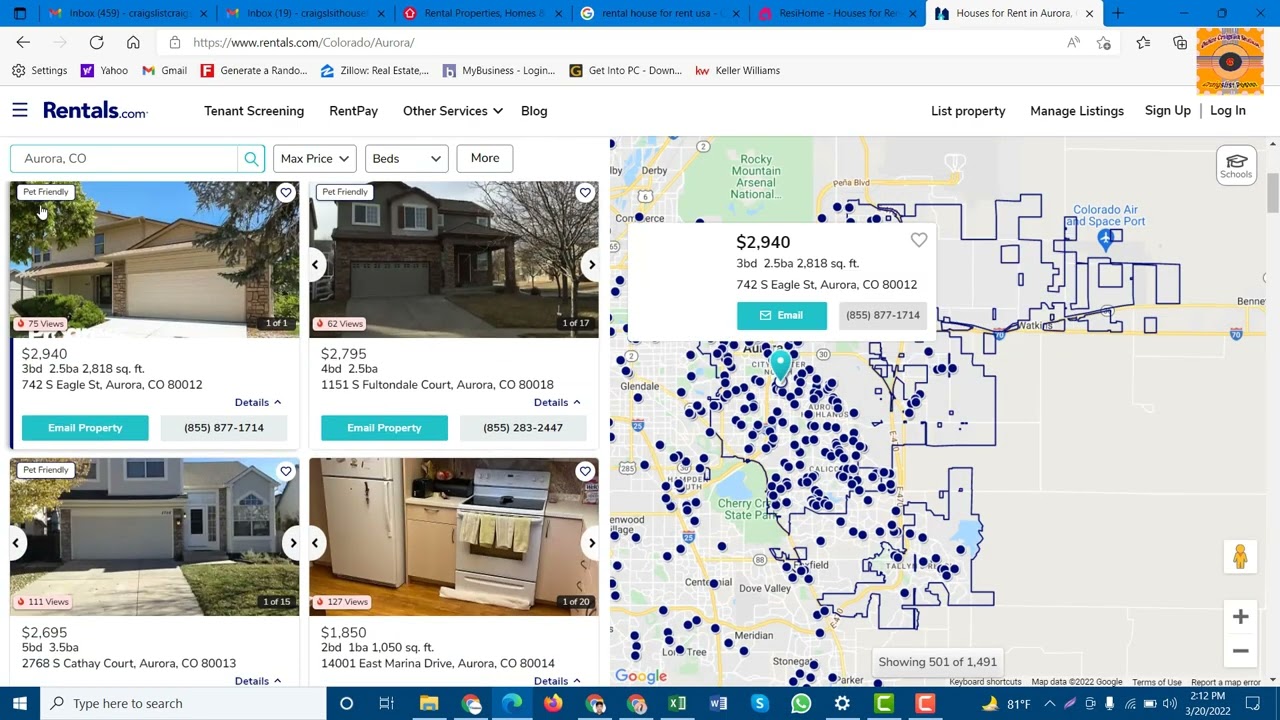A screenshot of a Rentals.com webpage showcasing various rental property features and tools. The webpage header displays navigation options such as "Tenant Screening," "Rent Pay," "Other Services," and "Blog" on the left, while "List Property," "Manage Settings," "Sign Up," and "Log In" are positioned on the right. 

The central feature of the page is an interactive map dotted with numerous blue markers, each indicating different rental listings. Among these listings, a prominent pop-up highlights a specific property: a spacious three-bedroom, 2.5-bathroom home spanning 2,818 square feet, located at 742 South Eagle Street, Aurora, CO, 80012, with a rental price of $2,940. The pop-up includes a green button labeled "Email" and a gray button displaying the phone number 855-877-1714 for direct inquiries.

On the left side of the screen, there are four thumbnail images of different house listings, each showcasing details such as price and bed/bath count, accompanied by "Email Property" and contact phone number options. Notably, one of the thumbnails at the bottom right provides a glimpse of a modern kitchen.

Additionally, the user interface reveals the operating system as Windows, and the presence of several open tabs at the top, with bookmarks for popular sites like Yahoo, Gmail, and Zillow, suggesting the user's active online session.